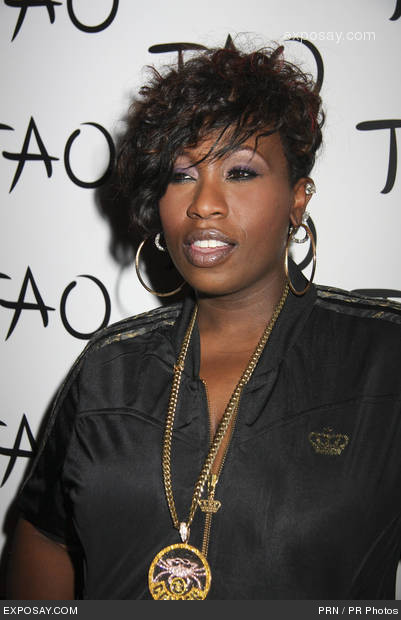This detailed image captures the iconic rapper Missy Elliott adorned in a black, silky shirt with a zipper partially unzipped to mid-chest. The left side of her shirt features an embroidered golden crown. Around her neck, she sports a gold chain with a circular medallion, displaying a design that resembles a purple and white crab, reminiscent of the Cancer astrological symbol. Missy accessorizes with prominent golden hoop earrings, complemented by smaller diamond-studded hoop earrings in a double-piercing. Her hair is styled short on the sides and back, fuller and curly on top, and swept across her forehead. She wears purple eye shadow and is captured smirking with her mouth open, showing her top teeth and a glimpse of her tongue. The backdrop is white with repeated black text letters "A-O-A-O", and the photo features the text "expose.com" in the top right corner as well as at the bottom along with "PRN/PR photos".